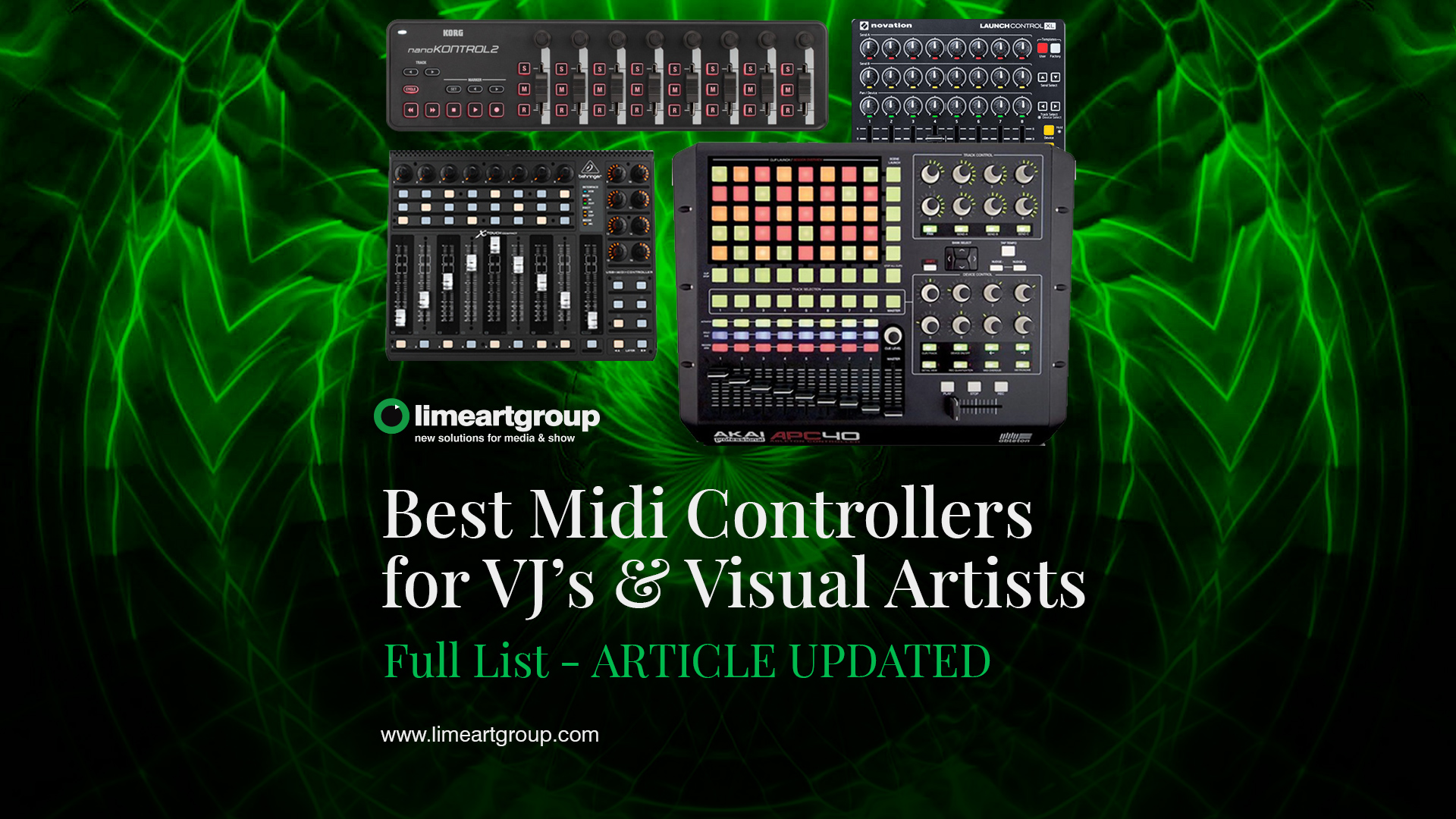This vibrant image appears to be an advertisement targeted towards VJs (video jockeys) and visual artists. Dominated by a sleek, black background accented with vibrant green lights and graphics, the focal point is an electronic device showcased at the top. This device, surrounded by multiple knobs and controls reminiscent of graphic equalizers, signifies its utility in sound and video processing. Below this central feature, in bold text, it reads, "Best MIDI Controllers for VJs and Visual Artists." Additionally, green text beneath this proclaims, "Full List Article Updated," with a small note of the website "Limeheartgroup.com" at the very bottom. The overall design suggests an engaging mix of audio and visual elements, catering to performers and tech enthusiasts alike.